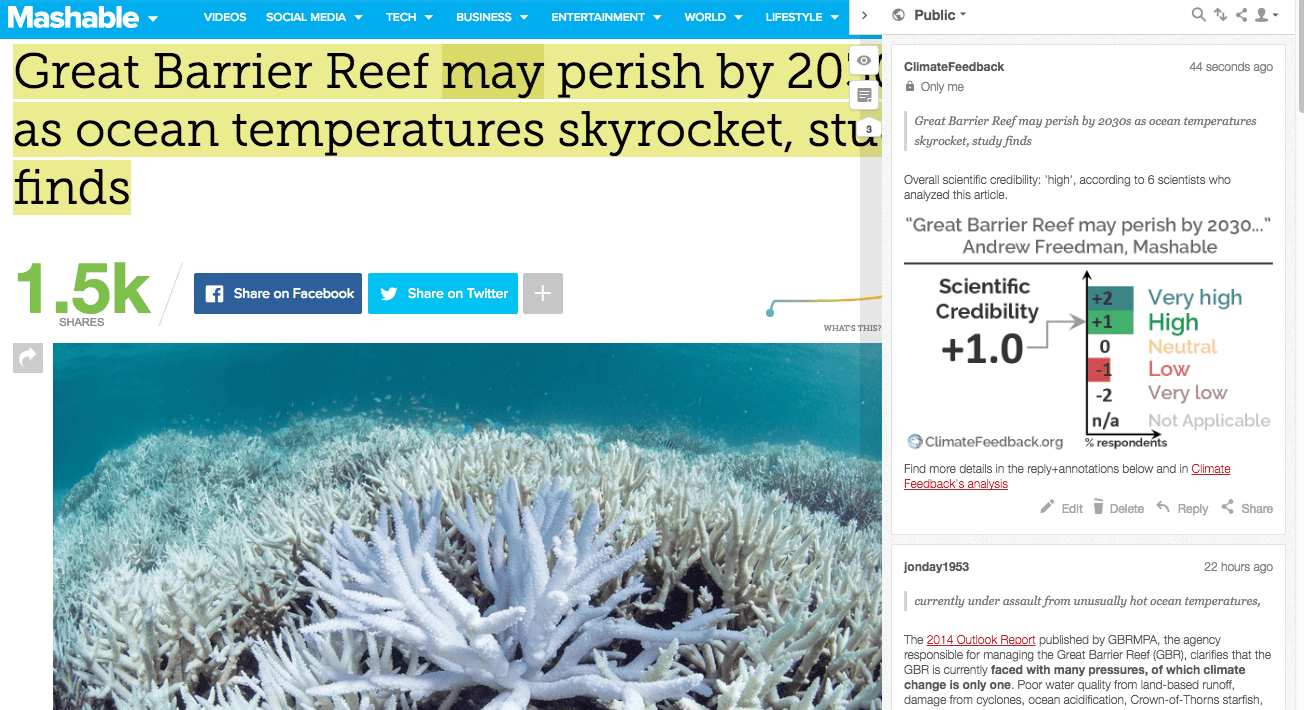This image is a screenshot from the website Mashable. At the top left, there is a blue navigation bar that reads "Mashable" in white text. To the right of the logo, the navigation tabs are labeled Videos, Social Media, Tech, Business, Entertainment, World, and Lifestyle. Below the navigation bar, there appears to be an article titled, "Great Barrier Reef May Perish by 2030 as Ocean Temperatures Skyrocket, Study Finds." This article has garnered 1.5K shares, with social media sharing options for Facebook and Twitter visible nearby.

The central part of the image features a photograph of an ocean floor scene. On the right side, a white sidebar with black text runs from top to bottom. This sidebar is labeled "Public" at the top, indicating it is part of the "Climate Feedback" section. It further details the article titled, "Great Barrier Reef May Perish by 2030," authored by Andrew Friedman. The image also indicates the scientific credibility of the article with a rating of plus 1.0, placing it on the high rating scale displayed within the image.